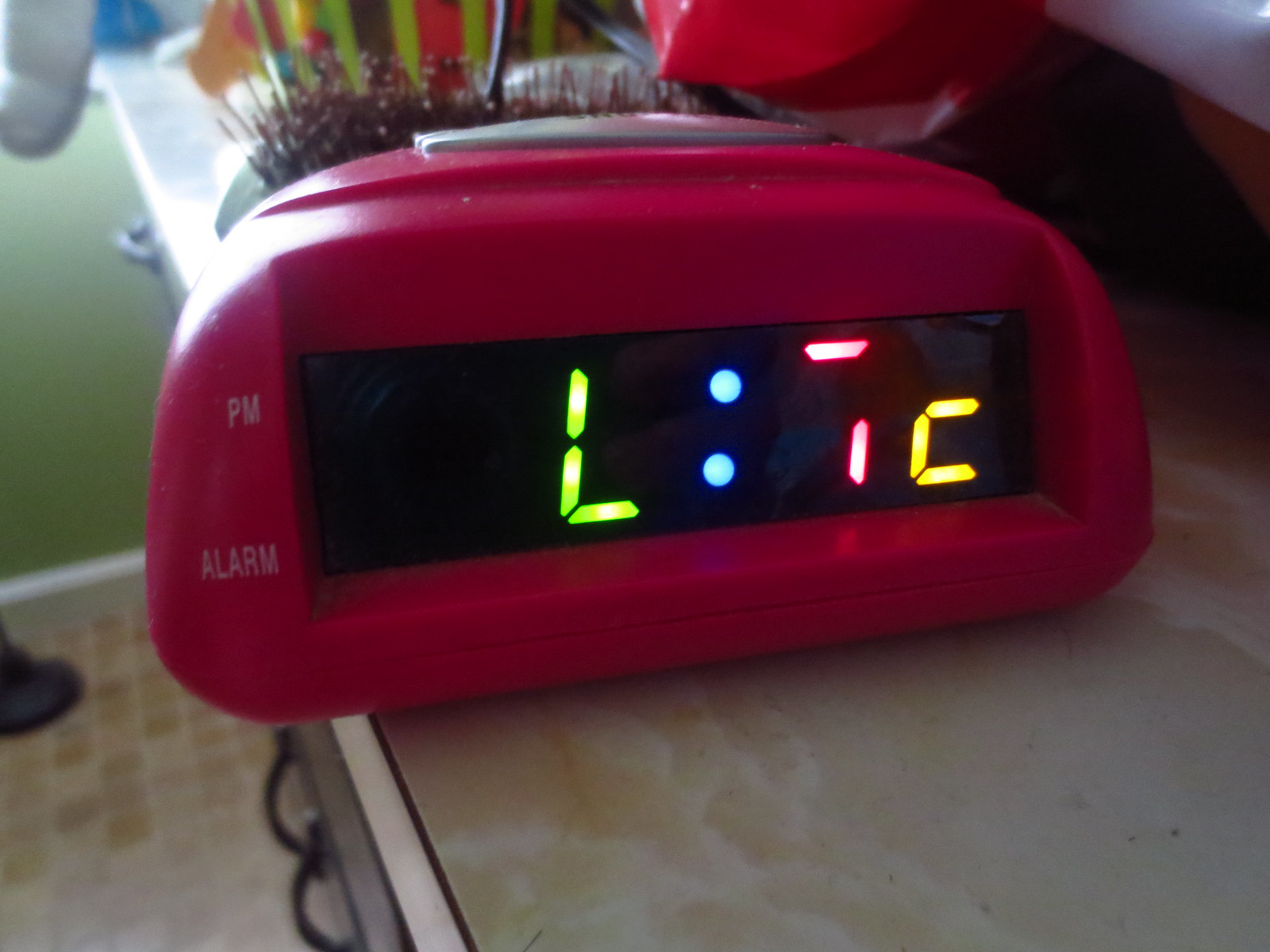The photograph depicts a close-up view of a malfunctioning red digital alarm clock. The clock is positioned on a gray and silver bedside stand or bathroom counter. The clock's display is not functioning correctly; it shows a sequence of characters: a green 'L', a blue colon (':'), the partial segments of a red '7', and a yellow 'C'. To the left of the display, the words 'p.m.' and 'alarm' are printed in white on the clock's frame. The background reveals brown tiled flooring, a sink, and a cabinet with drawers, suggesting the clock is placed in a bathroom. Additionally, other objects like a small plant, a round bowl, and possibly the base of a fan can be seen on the counter.